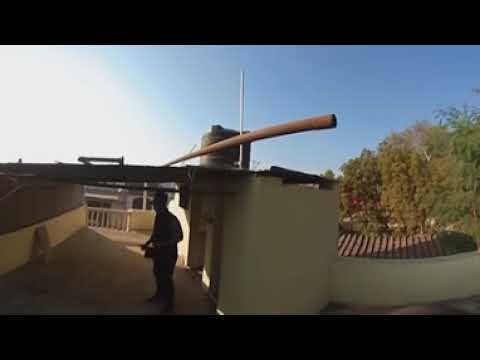The photograph depicts a man, possibly in a uniform, standing under the shadow of an awning attached to a short, guardhouse-like building with greenish walls and a reddish clay roof, featuring a cement structure with a flat roof. The awning, extending from the left structure to a smaller one on the right, mutes the man into a dark silhouette, suggesting he might be wearing a hat. The sky is clear and blue, with the sunlight casting long shadows, indicating the time of day is either early morning or late afternoon. Behind the man, a small white gate and a white fenced railing are visible, suggesting an entrance to a larger facility, potentially a military one. To the right, there is a walkway leading to more buildings and a row of trees, with some vegetation and laundry visible in the background, indicating the area is outdoors and spacious. Above the roof, a rusty pipe and another pipe structure can be seen, adding to the rustic ambiance of the setting.